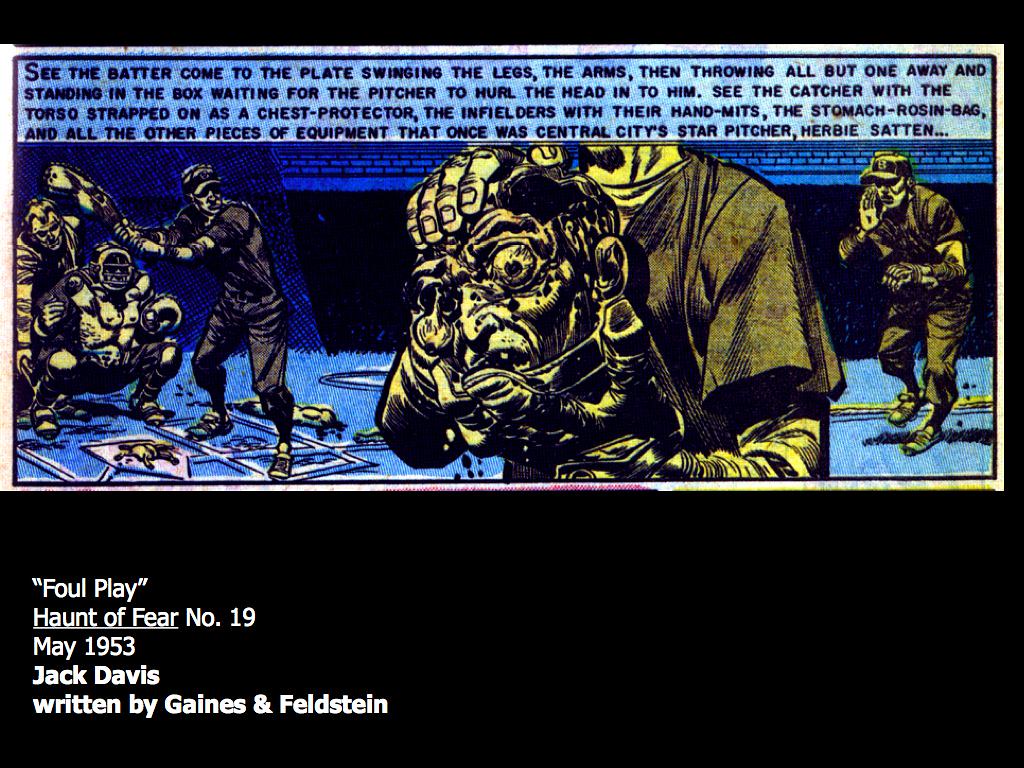This is an intricate pen and ink sketch reminiscent of newspaper or comic book art, featuring a surreal baseball game against a stark black background. Dominating the center-right is a grotesque figure holding a face resembling an Aztec symbol, with bulging eyes. At the bottom left, within the dark backdrop, the text reads "Foul Play," "Haunt of Fear number 19," "May 1953, Jack Davis," and credits the writing to Gaines and Feldstein. 

The topmost section of the image reveals a light blue rectangle with dark blue lettering that reads, "See the batter come to the plate swinging the legs, the arms, and then throwing all but one away and standing in the box waiting for the pitcher to hurl the head into him." This segment extends with further descriptions. 

In the baseball scene below, a man stands at home plate wielding a distorted bat, ready to hit what looks like a chicken carcass on the ground. Behind him, a catcher kneels in a traditional stance with a torso strapped to his chest protector, and an umpire stands just beyond. In the center of the image, a pitcher is dramatically depicted clutching a human head, its eyeball dangling, with a portion of the skull visibly chipped. Another character can be seen in the background, running the bases. This macabre and detailed image blends the ordinary with the horrific, creating a chilling yet captivating scene.